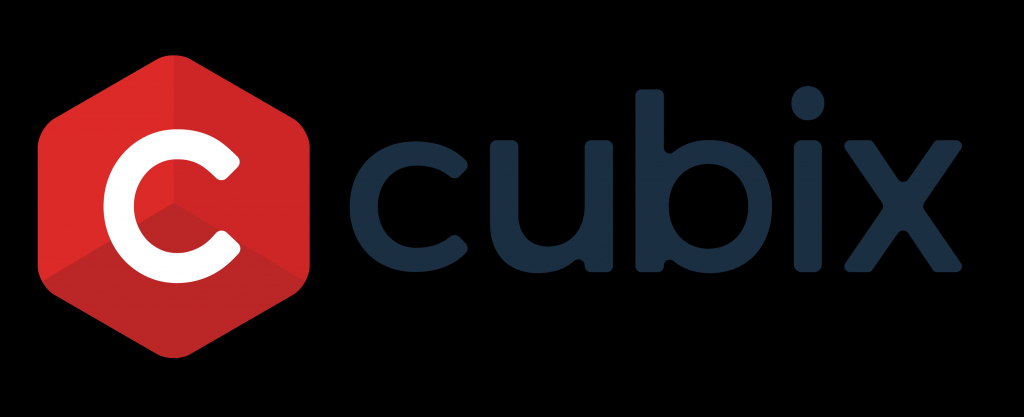The digital image depicts the logo of the company "Cubix" set against a black background. The logo is centrally aligned in a horizontal rectangular format. On the left side, there is a red octagon that resembles a three-dimensional cube with varying shades of red on its facets, giving it a striking depth. In the center of this red shape is a white, capitalized letter 'C' in a clean, sans-serif font, similar but slightly larger than the text to its right. 

To the right of this three-dimensional red shape, the company name "Cubix" is spelled out in all lowercase letters: C-U-B-I-X. These letters are gray and spaced slightly apart, maintaining a simple and straightforward alignment without any decorative elements. The entire design is minimalist, enhancing the readability and modern aesthetic of the logo. The black background encompasses the entire image, further emphasizing the clean contrast of the red, white, and gray elements.